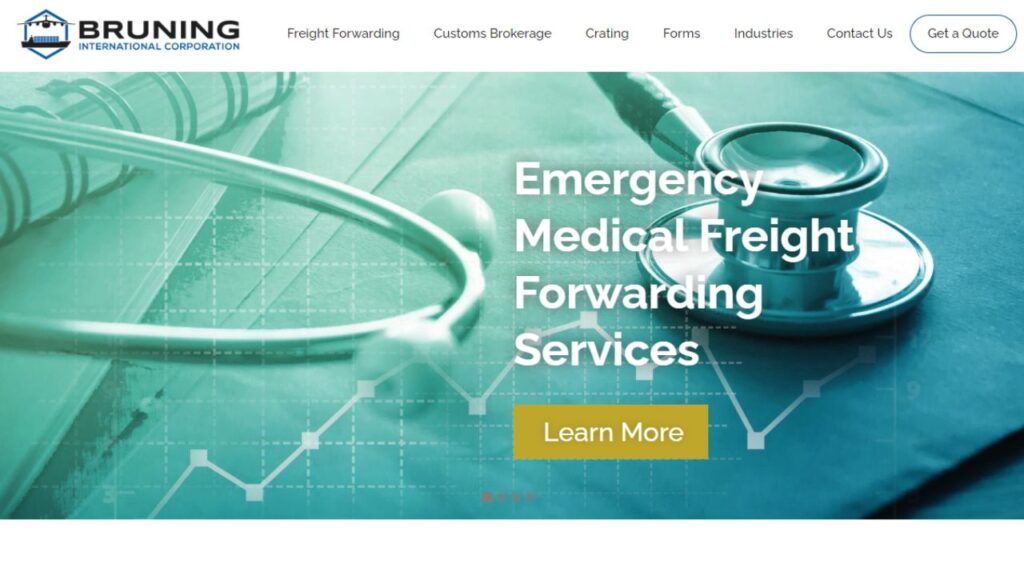This screenshot depicts a segment of the Bruning International Corporation website, which specializes in emergency medical freight forwarding services. The website's top section features a white background with the company's name on the left, accompanied by a distinctive hexagonal logo incorporating both an airplane and a cargo ship, symbolizing their expertise in multiple modes of transport. The navigation bar includes categories such as Freight Forwarding, Customs Brokerage, Creating Forms, Industries, and Contact Us, alongside an oval-shaped "Get a Quote" button.

Prominently displayed is a partial image of a stethoscope, with visible earpieces and chest piece, overlaid with a green and blue filter and a graphical element. White text across this image highlights the company's focus on "Emergency Medical Freight Forwarding Services." Below this text is a yellow button with the call-to-action "Learn More." The combination of elements underscores the specialized nature of Bruning International Corporation's services in the medical transportation sector.